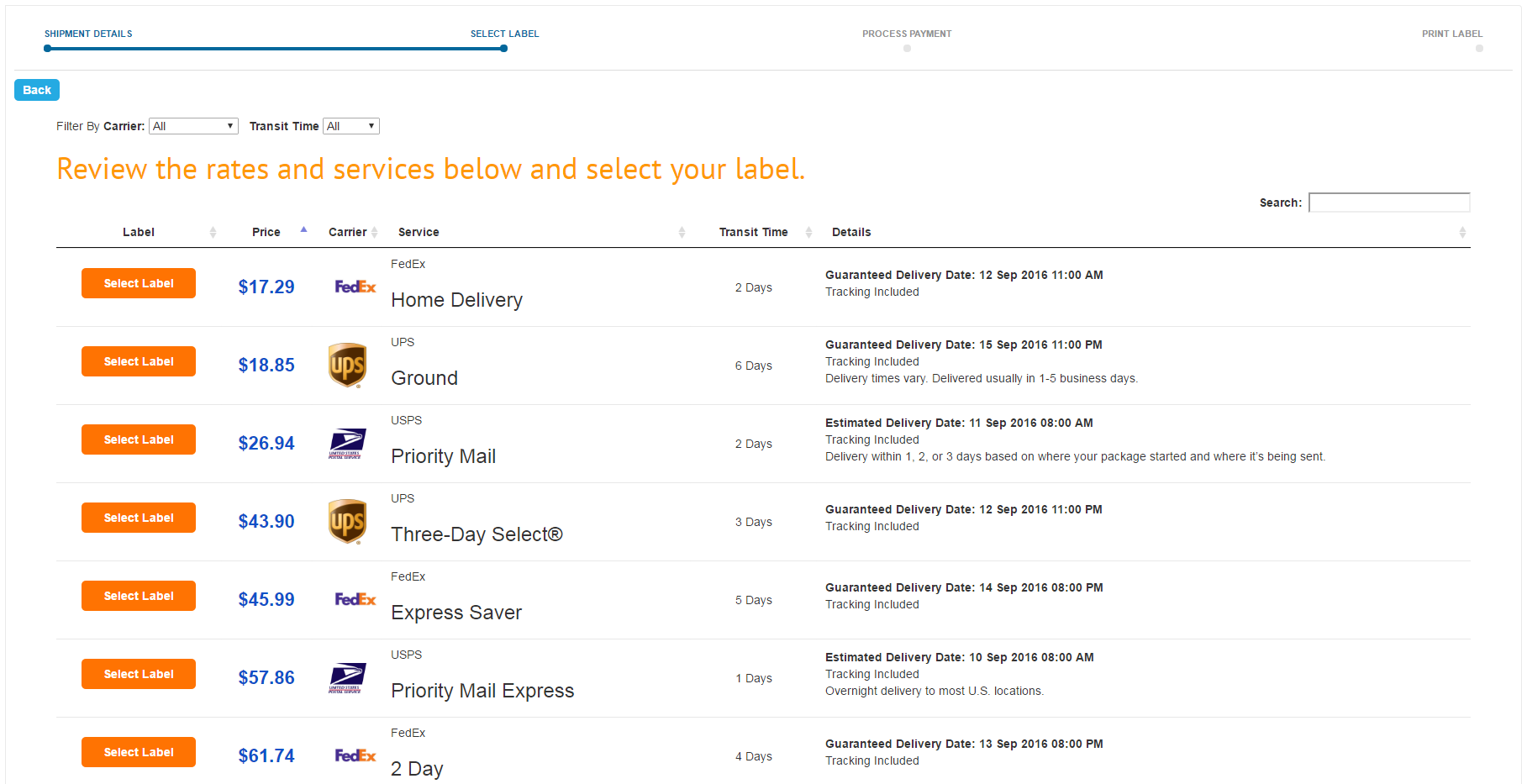Screenshot of a website displaying various shipping options sorted by price. At the top, there is a noticeable orange text that reads, "Review the rates and services below and select your label." Below this message, there is a menu for sorting the options. The list of shipping options, arranged from cheapest to most expensive, includes:

1. **$17.29 - FedEx Home Delivery (2 days)**
2. **$18.85 - UPS Ground**
3. **$26.94 - USPS Priority Mail**
4. **$43.90 - UPS 3-Day Select**
5. **$45.99 - FedEx Express Saver**
6. **$57.86 - Priority Mail Express**
7. **$61.74 - FedEx 2-Day**

Interestingly, the more expensive shipping options do not seem to offer significantly shorter delivery times compared to the cheaper ones, raising questions about their value for money.